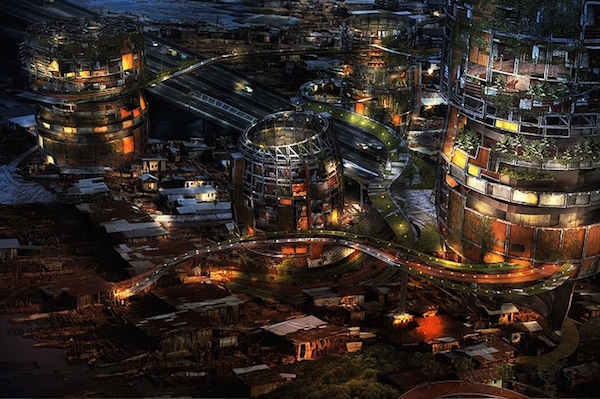This is an aerial photograph, likely taken by a drone, of a cityscape at night. The image prominently features a cluster of abstract, circular apartment buildings that are 10 to 15 stories tall. These buildings have terraces or decks adorned with flowers and some even have gardens. The roads surrounding these structures create a web-like pattern, with cars visible on a highway that appears to cross a bridge. In the far distance, there is a body of water, adding depth to the scene. The city is lit up, highlighting the vibrant colors of the platforms and the lights from the buildings' terraces. Beyond the main apartment buildings, there are scattered single-story shacks, giving the impression of a slum area. Train tracks weave between the buildings, adding an additional layer of complexity to the urban landscape.